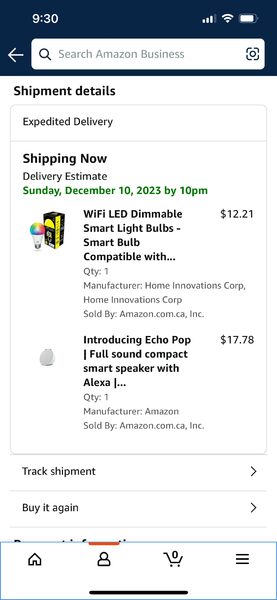The image depicts a webpage displaying an Amazon order tracking interface. The top of the page features a black header, including a search bar with the text "Search Amazon Business." In the upper right corner, there are icons indicating a full battery and full connection status. The time displayed is 9:30.

Below the header, the page is divided into several sections. At the top, bold text reads "Shipment Details," followed by "Expedited delivery" and the status "Shipping now." A green progress bar indicates the delivery estimate: "Sunday, December 10th, 2023 by 10 p.m."

The main section lists two products in the shipment:

1. **Wi-Fi LED Dimmable Smart Light Bulbs:**
   - Description: Smart bulb compatible with various devices.
   - Order quantity: 1 unit.
   - Price: $12.21.
   - Manufacturer: Home and Innovations Corp.
   - Seller: Amazon.com.

2. **Introducing Echo Pop - Compact Smart Speaker with Alexa:**
   - Visual: An image of a gray, round object, presumably the Echo Pop.
   - Price: $17.78.

Below the product information are two buttons: "Shipment Tracking" and "Buy it Again," both accompanied by right-facing arrows.

At the bottom of the page is a menu bar outlined in light blue with icons for Home, Profile (a person), Cart (indicating 0 items), and a three-line menu. Above the Profile icon, there is a small, red-goldish line.

The overall design uses a clear layout to provide detailed shipment information and facilitate navigation through various options and functionalities.